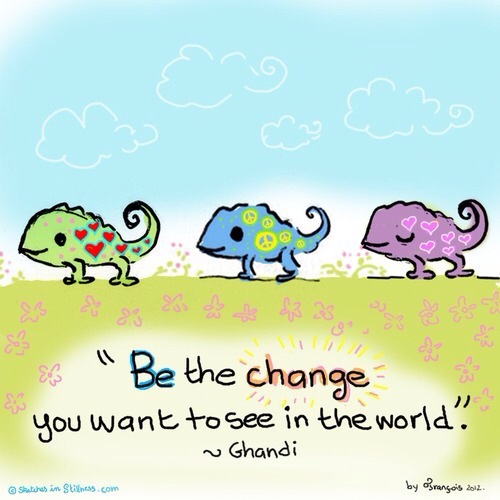The image depicts a charming, cartoonish scene with a blue, cloud-filled sky and a landscape of yellowish-greenish-brown grass. Three colorful lizards stroll from left to right, each adorned with distinct patterns: the first lizard is green with heart shapes, the second is blue with peace signs, and the third is purple, also with heart shapes. Above the scene, white, outlined clouds decorate the sky. A motivational quote at the bottom reads, "Be the change you want to see in the world - Gandhi." Additionally, the artwork credits "sketched by stillness.com" and "Francois, 2012" in smaller text at the lower left and right corners respectively.